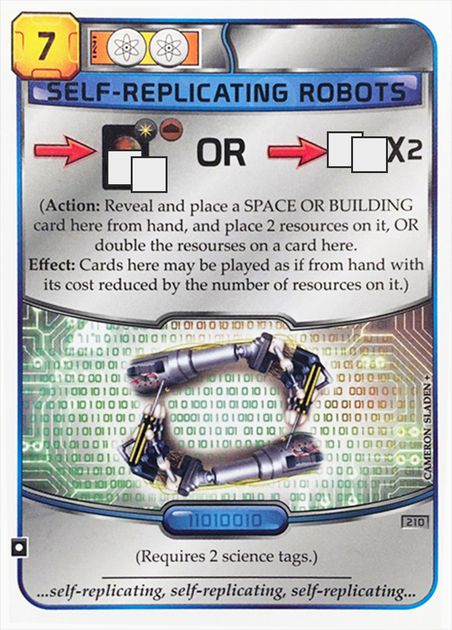The image depicts a game card, likely part of a tabletop or card game. In the top left corner, a yellowish-orange block prominently displays the number "7." To its right, two science symbols are depicted as double helixes within a similarly colored box. The top section extends into a silver stripe. Just below this is a blue banner with the text "Self-Replicating Robots" in black. The central part of the card features a gray background displaying an action and effect text: "Action: Reveal and place a space or building card here from hand and place two resources on it, or double the resources on a card here. Effect: Cards here may be played as if from hand with its cost reduced by the number of resources on it." Further down, robotic arms wielding screwdrivers are illustrated against a greenish-gray background with binary numbers. Beneath this, a circular frame contains a blue box with the binary sequence "11010010." The bottom section reverts to gray, stating, "Requires two science tags." The repetitive phrase "Self-replicating, self-replicating, self-replicating" appears at the very bottom of the card. Along the right edge, the name "Cameron Sladen" is written sideways.